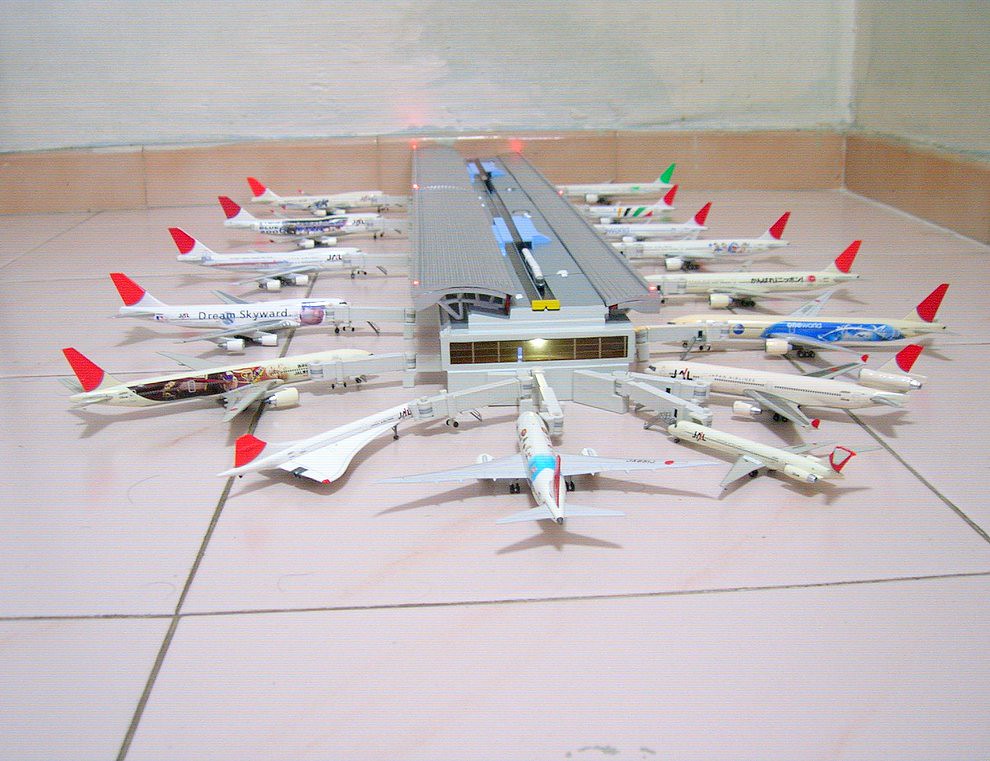The image showcases a detailed model of an airport set in the corner of a room with white walls and a peach-colored baseboard. The flooring consists of off-white tiles. Centrally positioned in the image is a miniature airport terminal with a gray roof adorned with red lights—three on each side—and blue objects on top. The terminal building features a horizontal window facing the viewer, illuminated from within. Surrounding the terminal are approximately 12 to 15 miniature airplanes, parked at their respective gates, primarily white with the distinctive feature of red tail fins, except for one green-tailed plane positioned at the back. The planes display various airline logos and markings, including "Dream Skyward," although most text is too small to decipher clearly. The planes are arranged facing the terminal with detailed walkways extending to the aircraft doors, enhancing the realistic depiction of a bustling airport scene.